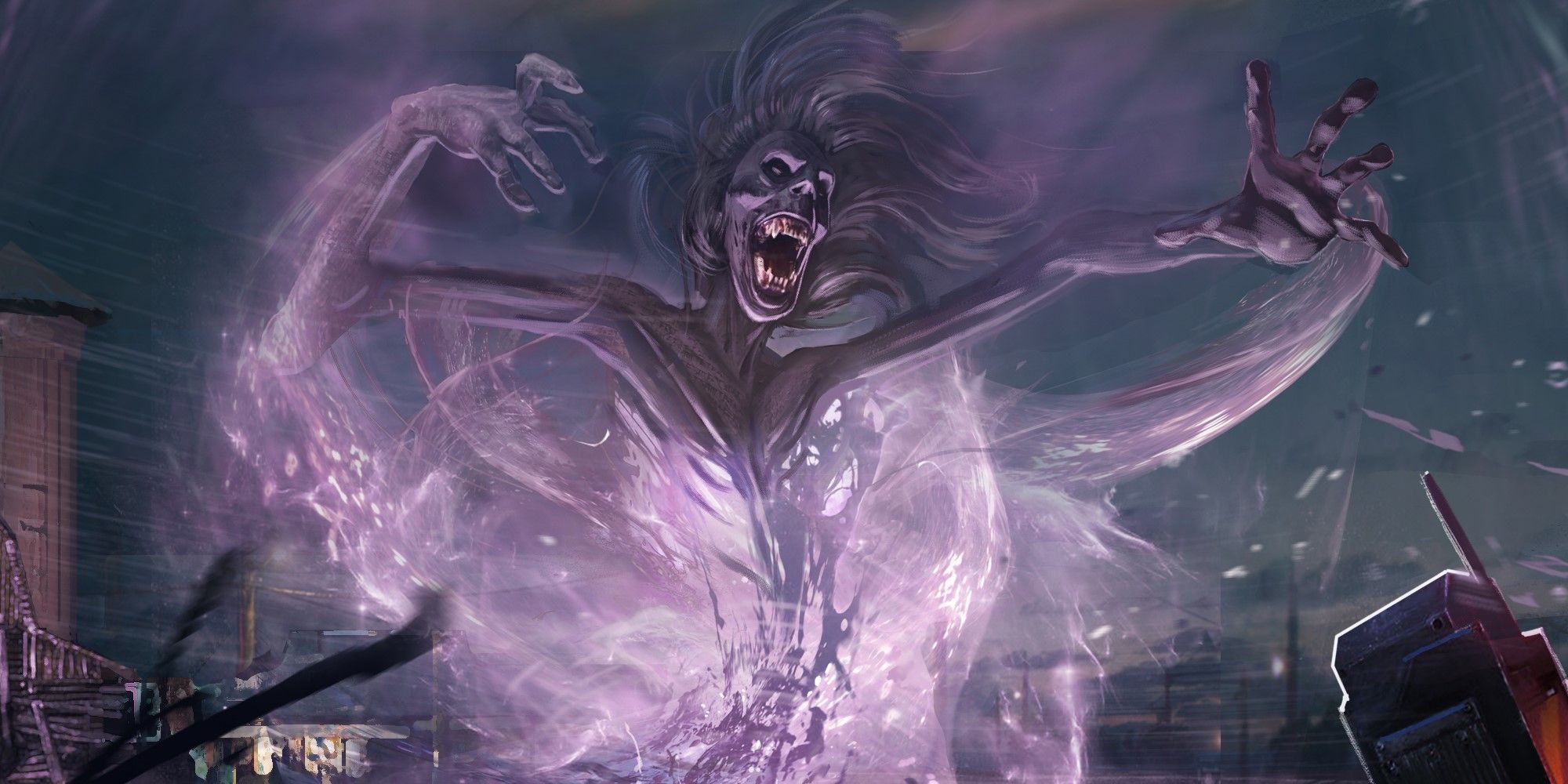The image is a highly detailed, computer-generated artwork, likely from a video game or as concept art for a movie like Ghostbusters. Set against a dark blue night sky, the scene is viewed from a first-person perspective, with a walkie-talkie-like device held in the bottom right corner. Dominating the center of the image is a colossal, ethereal creature.

This ghostly figure begins as a light purple, swirling vertical cloud at the bottom, which solidifies into a darker purple at the top. The creature has a muscular yet thin humanoid chest with extremely long arms ending in disproportionately large hands. Its open mouth reveals large, white fang-like teeth, and its face resembles that of a gorilla, complete with dark, sunken eyes. Flowing purple hair streams back from its head, adding to its intimidating presence.

The lower part of the ghost appears to be disintegrating into a vortex of purple and white light, giving it a spectral and wispy form. Surrounding the ghost is a whirlwind, enhancing its haunting appearance. The backdrop features a dark blue sky with hints of buildings and streetlights, grounding the scene in an urban environment. The creature appears to be captured in a ghost trap-like vortex, adding to its otherworldly and menacing aura.